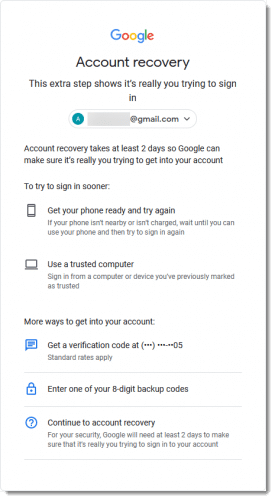In the image, a screenshot is displayed from a mobile device. At the top, the familiar Google logo is shown in its iconic multicolored letters, followed by the text "Account Recovery." Below, there is a message indicating an additional verification step to confirm the user's identity for sign-in purposes. 

For privacy, the user's email address has been obscured with a gray rectangle, though a teal circle with a capital letter "A" is partially visible. Despite the masking, part of the email's suffix that reads "@gmail.com" is apparent.

The message further informs that the account recovery process takes a minimum of two days for Google to ensure the legitimate owner is attempting to regain access. To expedite the process, two options are provided: using a phone or a computer. The instructions detail:

1. **Get Your Phone Ready**: If the phone is not immediately available or charged, wait until it is accessible and then retry the sign-in.
2. **Use a Trusted Computer**: Sign in using a computer or device previously marked as trusted by the user.

Additionally, there are more options to regain account access, highlighted by a speech bubble icon. It suggests obtaining a verification code and mentions entering one of the user's eight-digit backup codes as an alternative. It concludes with an option to "Continue to Account Recovery."